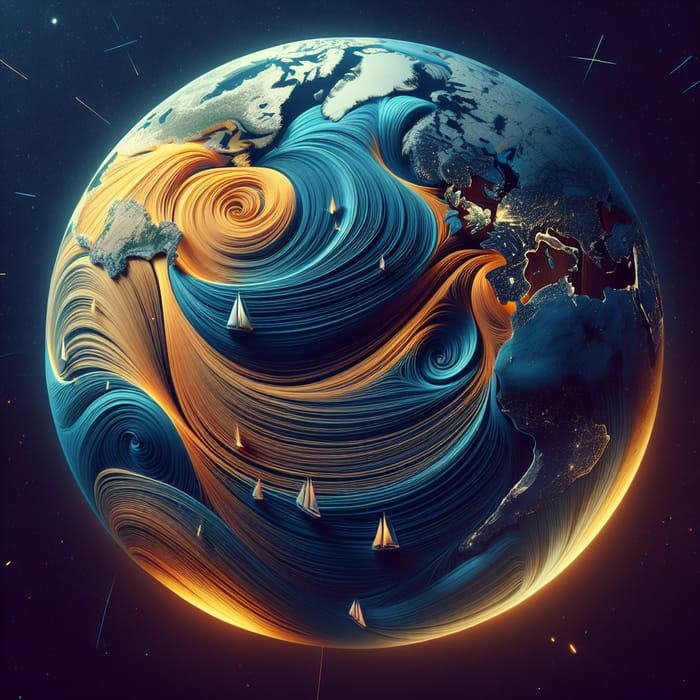The image appears to be an AI-generated, futuristic depiction of Earth, set against a striking ombre background that transitions from purple at the bottom to blue at the top. The central focus is a round, globe-like structure adorned with intricate swirls of blue, yellow, and orange, giving it an ethereal, otherworldly feel. At the bottom of the globe, the light, possibly representing the sun, breaks through in a radiant golden-orange hue. Scattered across the surface are several sailing ships, adding a sense of dynamic movement. The right side of the globe features detailed landmasses, including a recognizable outline of Africa and what appears to be a cityscape illuminated by minimal lights. Higher up, the globe shows continents seemingly encased in ice, with clouds hovering above. Surrounding the globe are representations of stars and possibly comets or asteroids, enhancing the celestial atmosphere of the image. The background is further detailed with emanating white lines, adding depth and complexity to the overall scene.